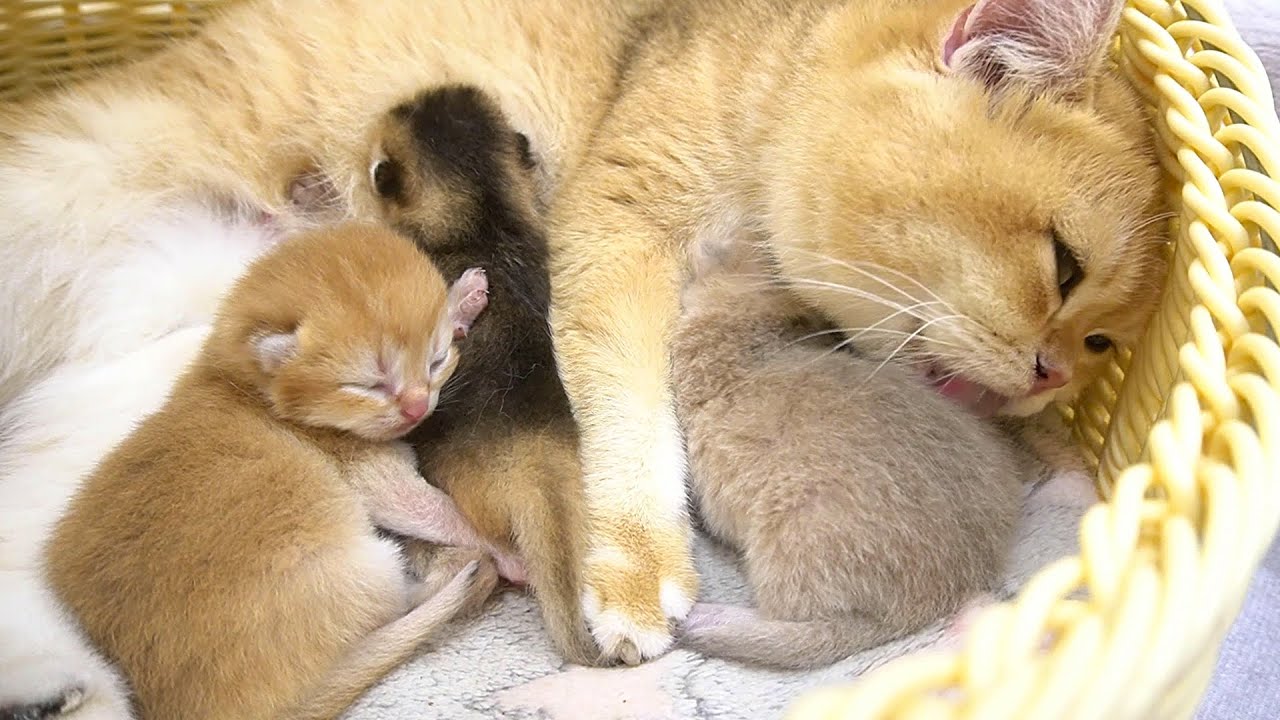The photograph captures a serene scene of a mother cat and her three kittens nestled in a light-colored basket lined with blankets. The mother cat, predominantly white with patches of golden and black fur and possessing a characteristically flatter face, is lovingly licking one of her kittens. This particular kitten, located on the right, is a mix of light brown and gray shades, although its head isn't visible, as it is either nursing or sleeping.

Adjacent to this kitten, in the middle of the basket, is another kitten with striking yellow-orange fur and distinct black markings on its back and head. This kitten appears to be nursing, its face obscured as it seeks nourishment. On the leftmost side, an orange kitten with closed eyes is peacefully sleeping, partially resting atop the black-backed kitten that is nursing. The tranquil family scene is bathed in the soft, natural light filtered through the room.